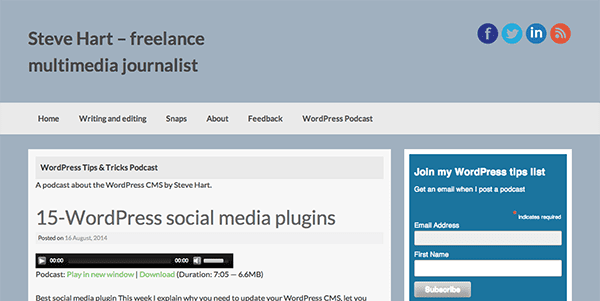At the top of the webpage, a gray navigation bar stretches horizontally across the screen. On the left side of this bar, black text reads "Steve Hart - Freelance," with "Hart" spelled H-A-R-T. Directly underneath this text, it identifies Steve Hart as a "Multimedia Journalist." 

In the center of the gray bar, there is a blank space. Positioned in the upper right corner, social media icons are displayed, including Facebook, Twitter, Indeed, and a red circle containing a Wi-Fi symbol.

Beneath the gray bar, there is a lighter gray colored navigation menu featuring black text with various options: Home, Writing and Editing, Snaps, About, Feedback, WordPress Podcast.

The background transitions into a grayish-blue color. On this background, a white block appears on the left with a corresponding blue block on the right. The text over these blocks announces "WordPress Tips and Tricks Podcast 15 WordPress Social Media Plugins," accompanied by an audio clip for listeners.

On the right side, a subscription form invites visitors to "Join my WordPress Tips List," with fields provided to enter a first name and email address.